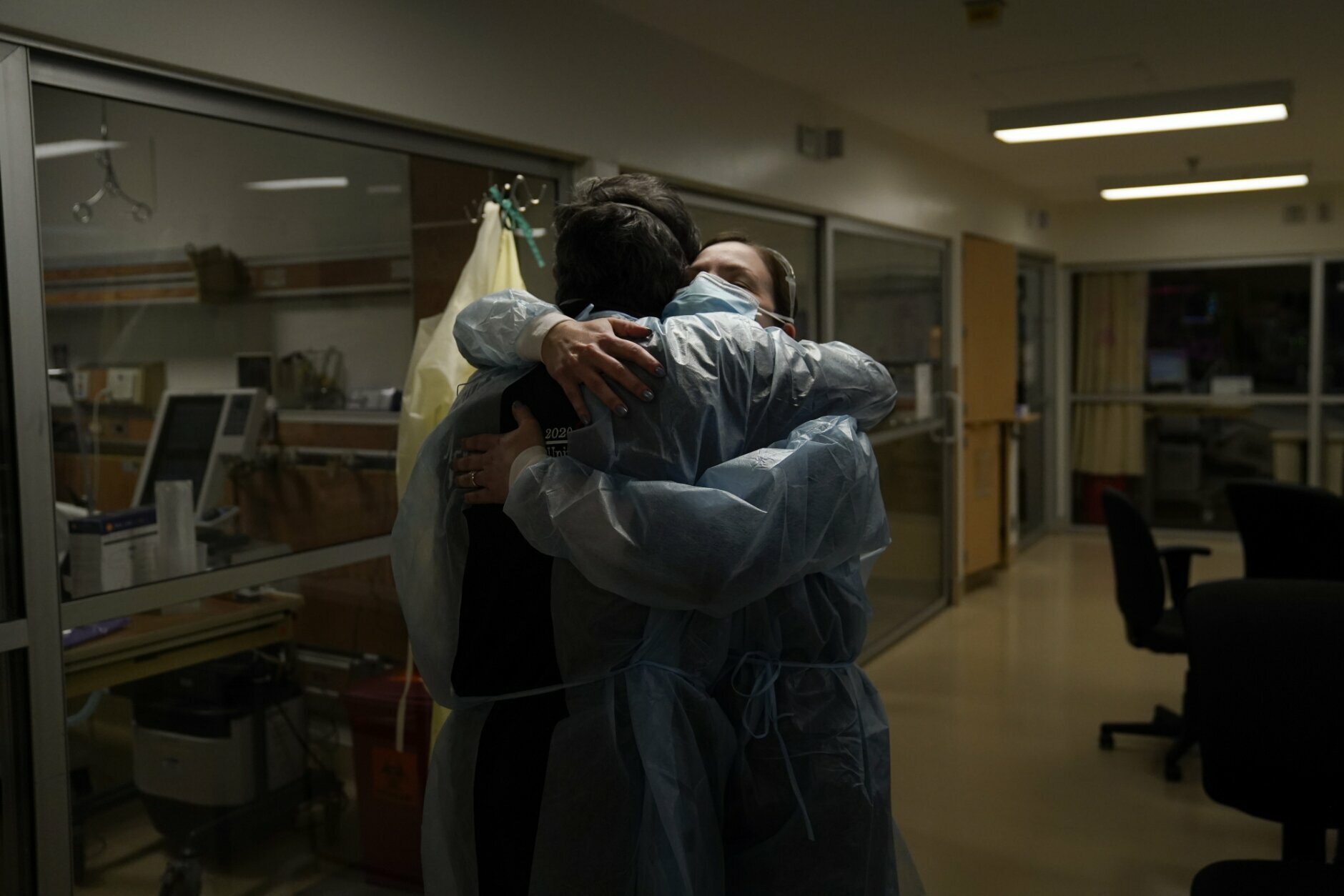This image captures an intense and emotional moment in a dimly lit hospital setting, possibly in an emergency or surgery recovery area. Two healthcare professionals, clad in blue plastic protective coverings and face masks, are embracing each other tightly in what appears to be a significant moment of relief or support, perhaps after a challenging procedure. They stand in a large hallway illuminated by fluorescent light tubes stretching across the white ceiling.

The hallway features numerous sliding glass doors and large windows that provide a view into various rooms filled with medical equipment, office chairs, and computers. You can make out an operating table and other surgical instruments in an adjacent room, as well as a yellow IV bag and other hospital apparatus. The scene is filled with both tension and relief, capturing a rare personal moment of connection amid the clinical efficiency of the hospital.